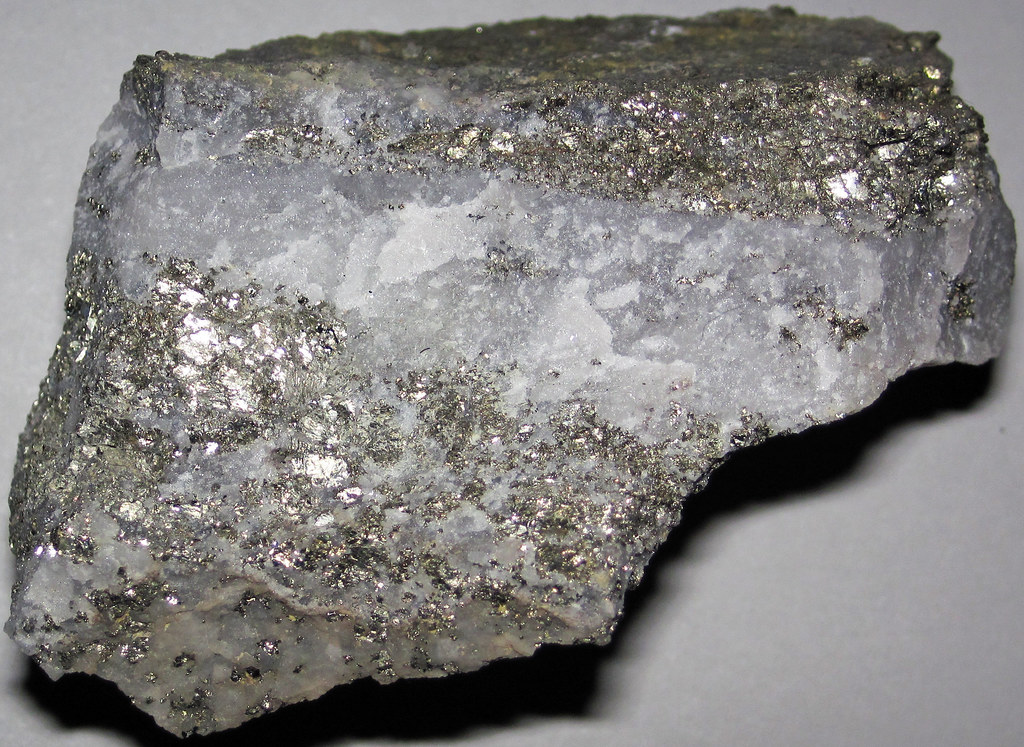This image features a slab of rock with jagged, sharp edges resting on a light gray surface, casting a dark drop shadow. The rock is predominantly gray, with a distinctive cloudy strip of light gray or milky gray quartz running across its center. The surface of the rock is studded with small, silver-colored metallic shards and tiny fragments that give it a subtle sparkle, reflecting light and adding a touch of shimmer. The top of the rock is flat, but the sides are smooth yet rough and jagged at the edges, enhancing its rugged appearance.